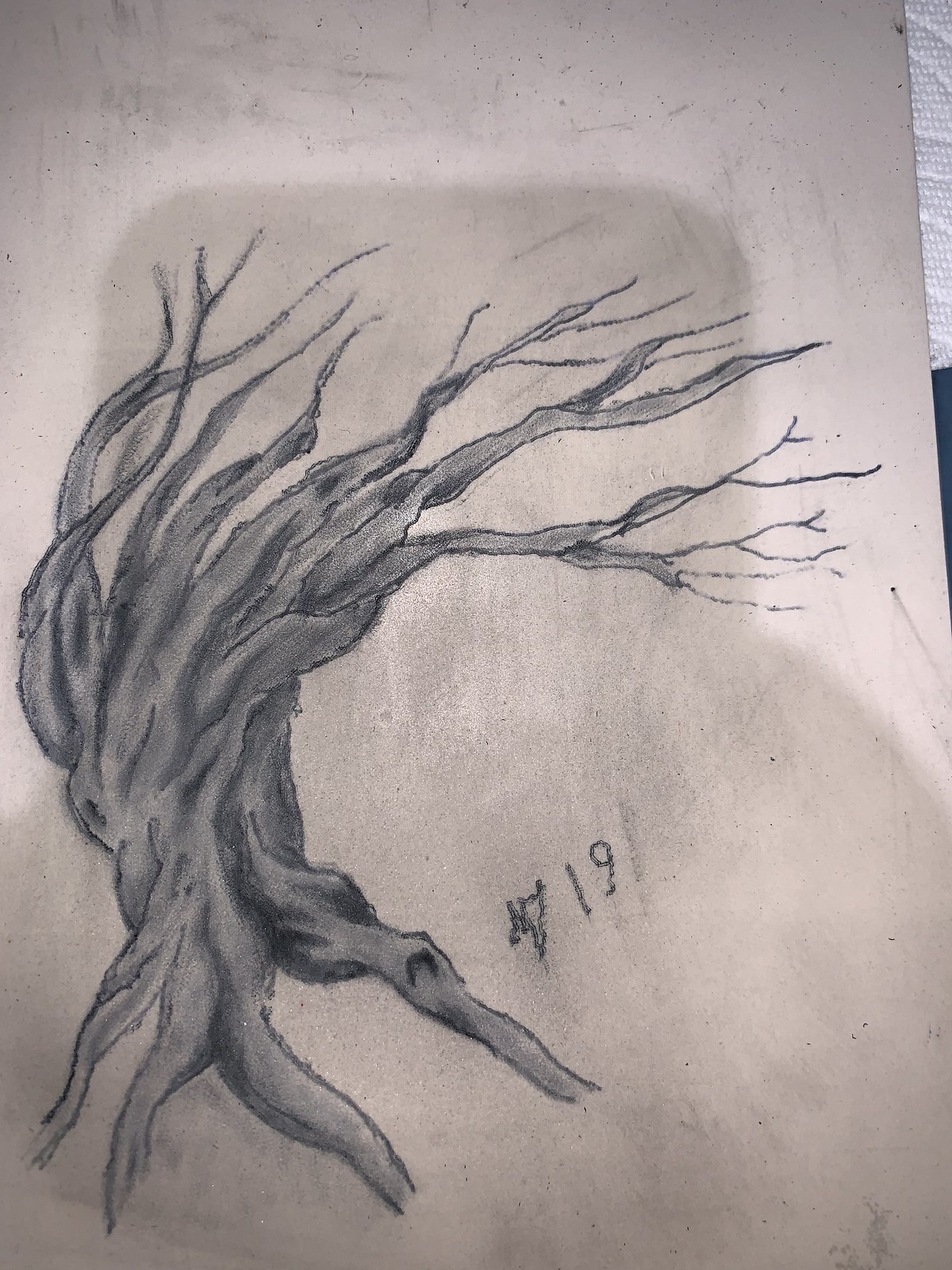The photograph captures a detailed drawing on dark cream-colored paper, possibly intended to be a lilac gray surface. The artwork showcases a solitary, heavily shaded, gnarled tree, which appears to be done primarily in pencil or perhaps dark crayon. The tree is centered towards the left side, with its twisted trunk starting at the bottom left corner and its thick, wind-blown branches extending upwards and to the right. The intricate depiction includes four prominent roots, one with a hole, suggesting depth and perhaps a hidden critter's abode. The number '19' is clearly visible beside what appears to be the artist's initials, 'M' and possibly 'J.' A noticeable shadow, likely of the photographer holding a phone, is cast upon the image, adding to the photograph’s narrative. No grass or additional elements are featured, focusing all attention on the solitary, expressive tree.